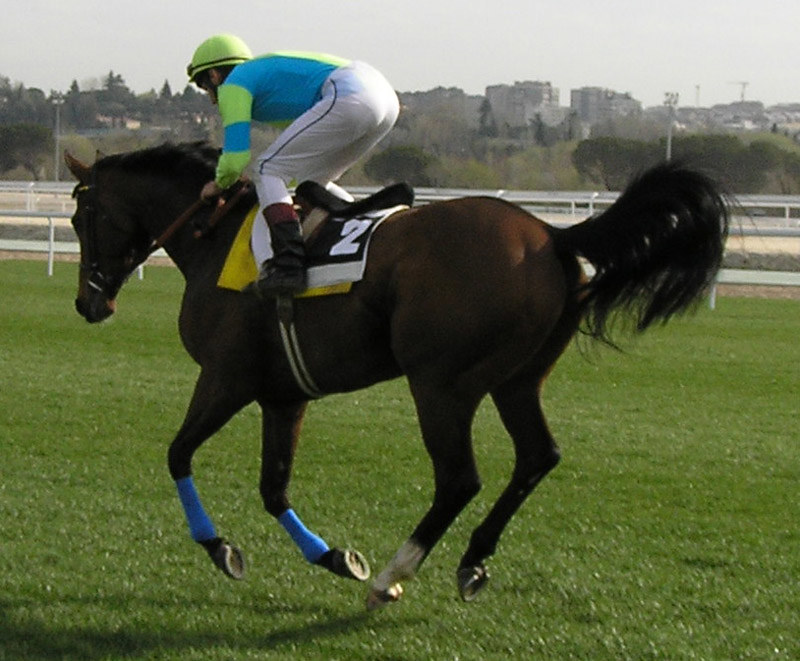The image depicts a jockey in an upright, crouched position, cantering a dark bay racehorse with a black tail on a lush, smooth grass turf track. The horse, with all four legs off the ground, displays bright blue polo wraps on its forelegs and a white stocking on its left hind leg. It bears a yellow and black saddle with the number two emblazoned on it. The jockey is adorned in white riding pants, black riding boots featuring a brown leather strip at the top, and a blue jersey with bright green stripes on the sleeves. His bright green helmet features a black band. Surrounding the track is a white picket fence, with grassy hills, gray buildings, and trees forming the backdrop.